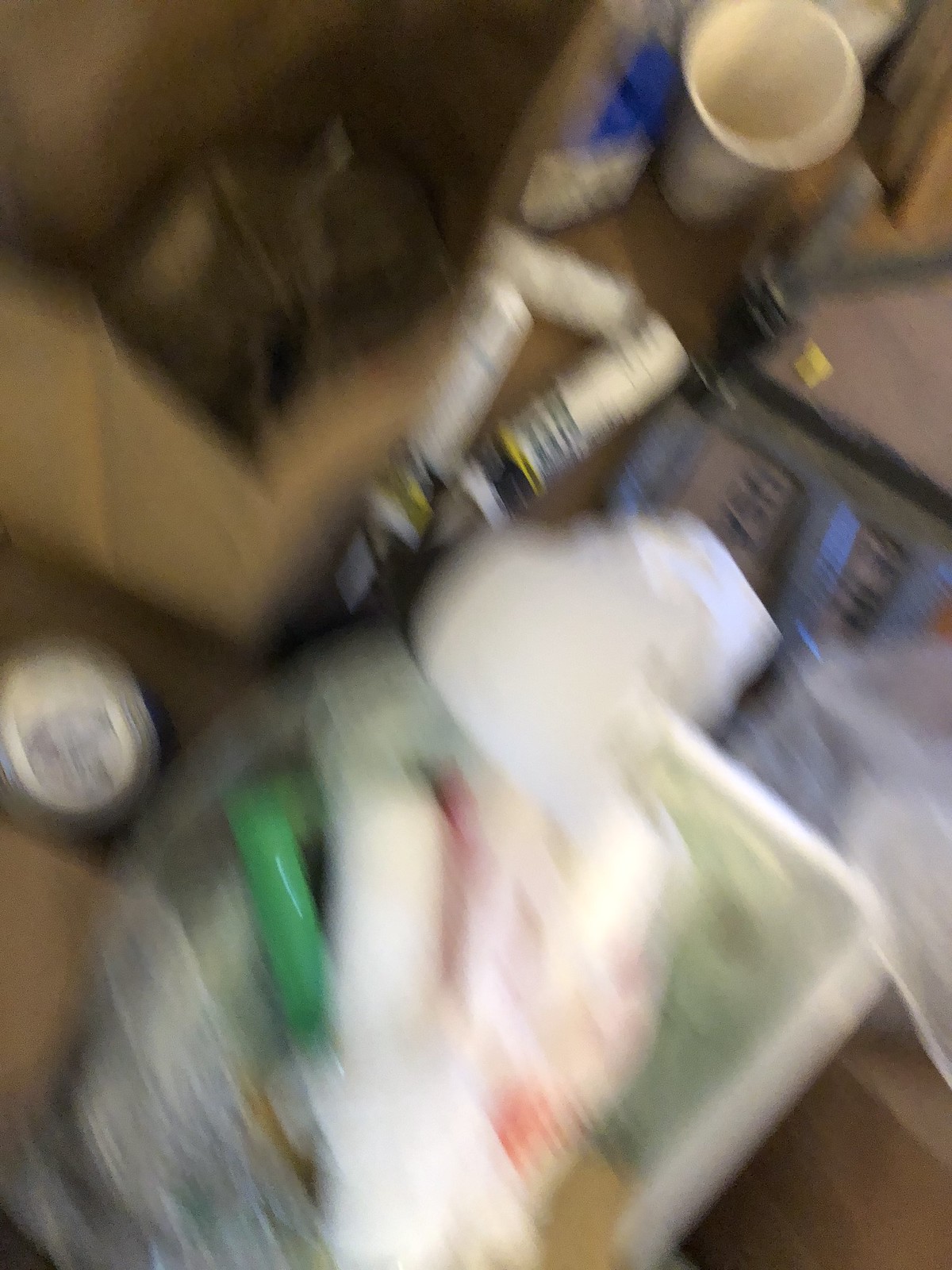This image is extremely blurred, depicting a cluster of various objects, making it difficult to discern specific details. Dominating the lower half of the photo is a plastic-like sheeting or packaging material that obscures much of the view. To the left, there is a smaller object with a metallic cap. Slightly above this capped object, a small electronic device with faint displays can be seen. At the center of the image, there are three cylindrical objects resembling shotgun shells. The upper-left corner is occupied by what appears to be a crumpled paper bag. An off-white, possibly styrofoam or paper serving cup is also visible. All these items rest on a brown surface, likely a countertop or table.